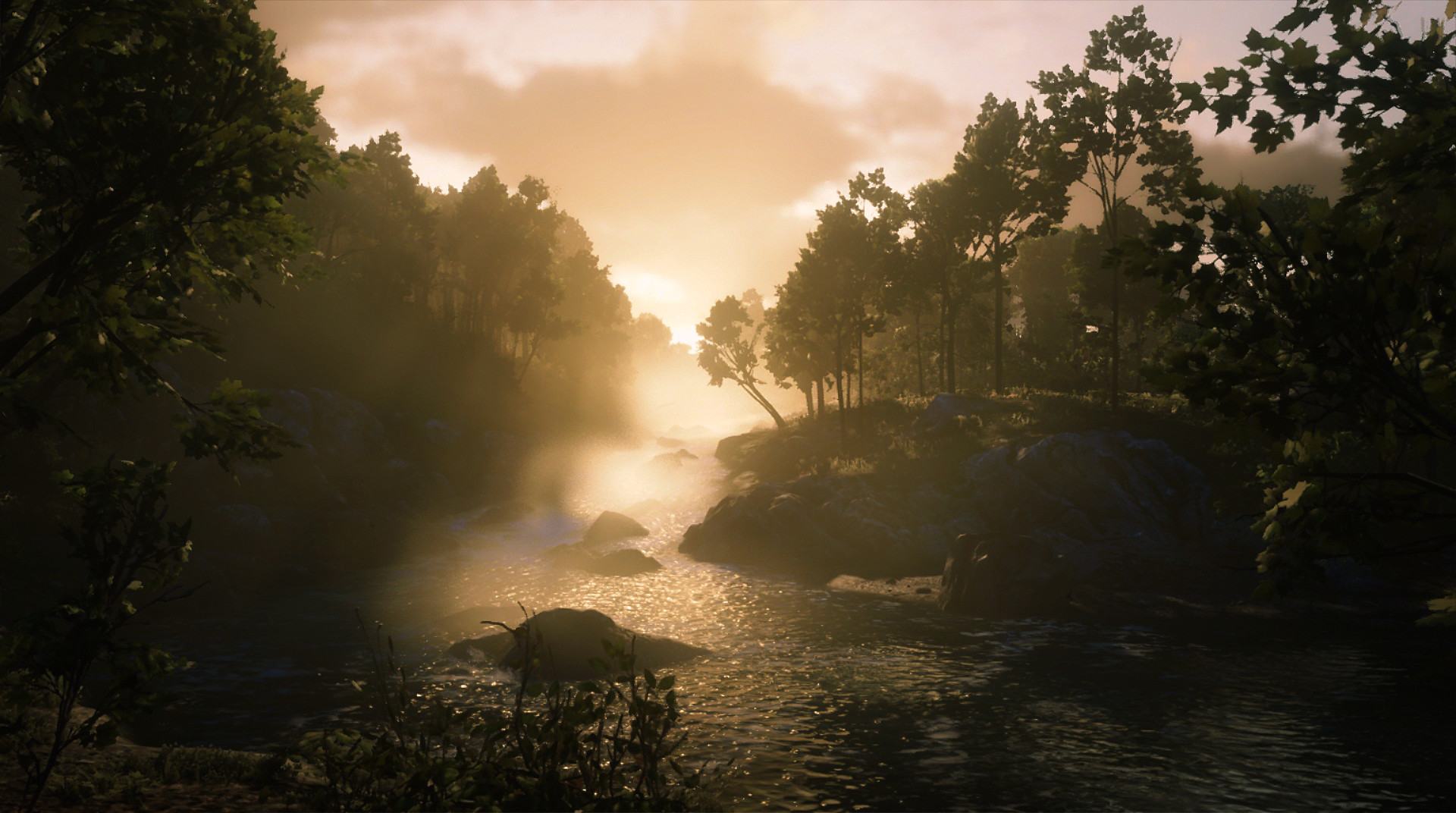This captivating outdoor photograph showcases a serene stream, likely an offshoot of a river, with visible flowing water. The scene is bathed in the ethereal light of either dawn or dusk, imparting a striking pink hue that reflects on the water and suffuses the sky with a beautiful pink-purple gradient. Wisps of fog roll gently across the water, enhancing the misty ambiance, while dark, mist-shrouded clouds linger above.

In the stream, large boulders and smaller black rocks punctuate the water's path, adding a rugged texture to the scene. Greenery abounds around the stream, with bushes and trees densely populating the area, their reflections visible in the calm sections of the water. Scattered amidst the lush vegetation are a few delicate flowers, dotting the landscape with subtle splashes of color. Together, these elements create a tranquil and picturesque natural setting.